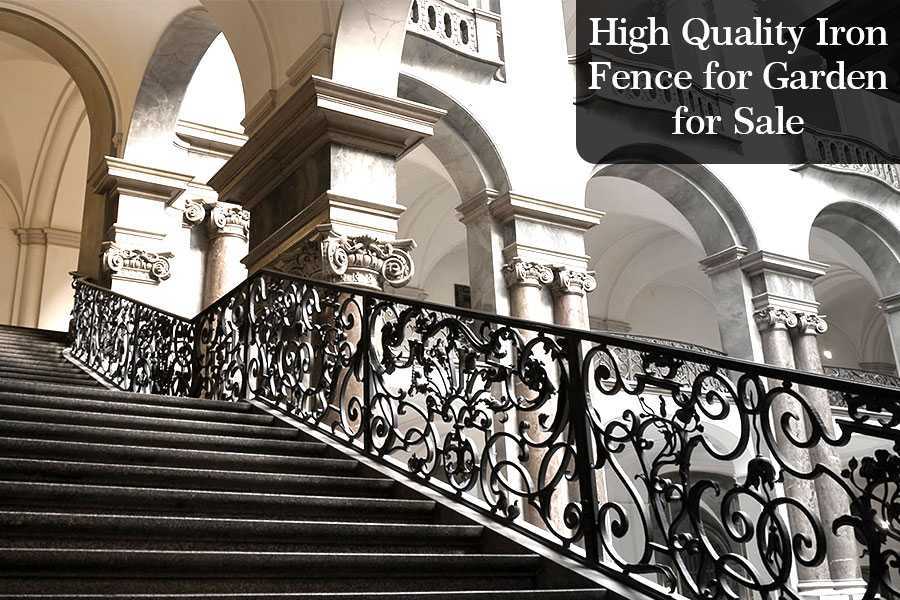For sale: Exquisite, high-quality iron fence ideal for garden enhancement. This detailed poster features a photograph of the ornate iron structure, beautifully set against a backdrop of classical architecture. The background reveals grand columns and arches, epitomizing timeless elegance. A wide stone staircase ascends gracefully, highlighted by the iron fence that extends from the lower right to the upper center of the image, creating a dynamic perspective. The intricate designs of the banister showcase the craftsmanship and sophistication of the ironwork, making it a stunning addition to any garden or outdoor space.